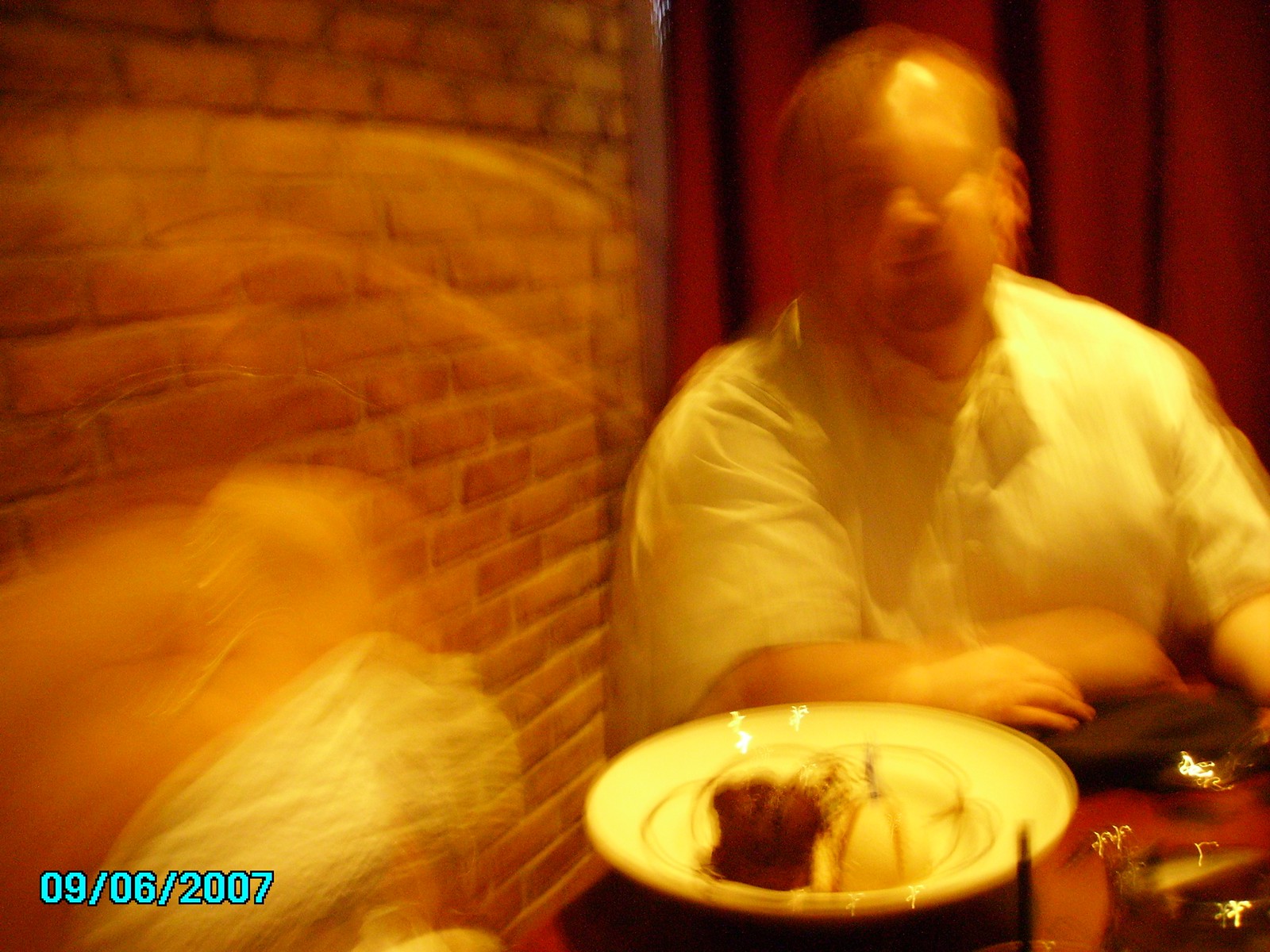In the image, there is a person seated at a table in what seems to be a restaurant environment. The left side of the image shows a wall, while behind the man, there is a red curtain. The table in front of him features a plate holding what appears to be a decadent dessert, possibly ice cream and a slice of chocolate cake. The man is dressed in a simple white long-sleeve shirt with the sleeves rolled up. He has a bald or nearly bald head, though the image is slightly blurred, making it difficult to be certain. To the right, there is a partially visible figure, but only their body is somewhat discernible. The date "09.06.2007" is also visible in the image.